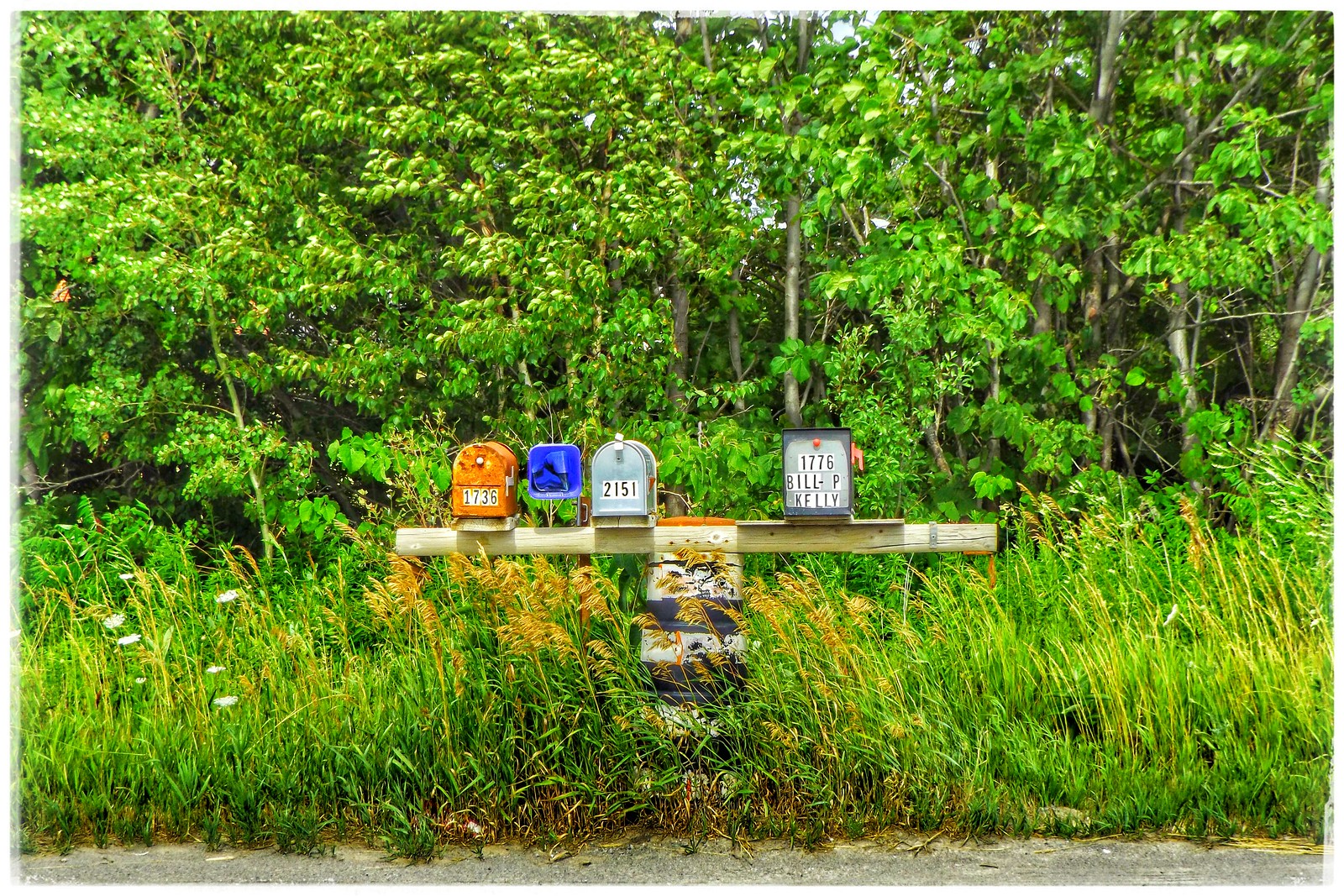This outdoor photograph, taken during the daytime, features an eclectic arrangement of colored mailboxes atop a rustic wooden stand. The stand, made of what appears to be gray and white barrels stacked vertically, supports a horizontal light brown post. On this post rests a series of mailboxes, each uniquely colored and numbered. From left to right, the mailboxes include a rusted orange box labeled 1736, a blue box intended for newspapers, a silver metal mailbox with the number 2151 and a red flag, followed by a notable gap suggesting a missing mailbox. Another distinctive mailbox on the right is square-shaped with a red knob and labeled 1776, Bill-P Kelly. Surrounding this mailbox stand are tall strands of green and golden-yellow grass, interspersed with some tall white wildflowers on the left. The scene is framed by a slim, grayish road visible at the very bottom, peeking through the grasses. In the background, a row of thin but tall trees with green leaves completes the picturesque setting, creating a serene and lightly wooded backdrop.